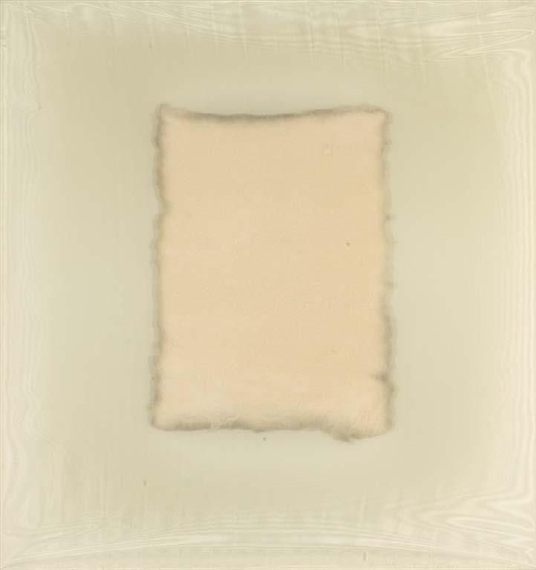The artwork is an abstract mixed-media creation, nearly square in shape, featuring a background that appears to be composed of white or off-white aged fabric or canvas, with visible brushstrokes and subtle shades of cream and pale green. This gives it a slightly weathered and textured look. Centered within the piece is a vertical, rectangular shape reminiscent of a piece of burned or torn paper. The rectangle is outlined by uneven, faded, rippled edges with a muted, graying, and ragged appearance, suggesting it has weathered over time. The interior of the rectangle is a soft, solid, light beige or very faint peach color, enhancing the overall impression of faded antiquity. No text or markings are present, adding to its minimalistic and enigmatic nature.